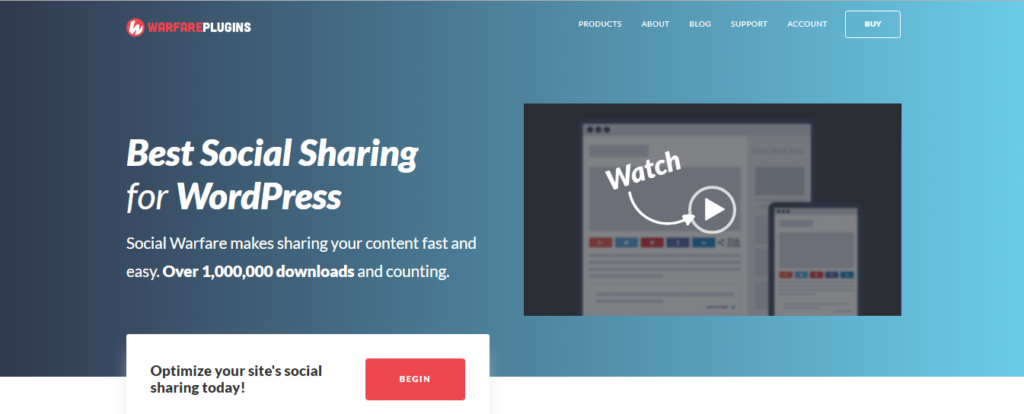This screenshot captures a promotional section of a website designed to help users share and promote content on WordPress efficiently. The layout is a long, horizontal rectangle that features a gradient blue background, transitioning from dark blue on the left to baby blue on the right. 

In the top left-hand corner, the branding is clearly displayed with "Warfare" in bold red text followed by "Plugins" in crisp white text. Accompanying this text is a distinctive logo: a red circle with a tilted white "W" inside. 

On the top right-hand corner, a navigational menu in all-caps white text includes the following options from left to right: "PRODUCTS," "ABOUT," "BLOG," "SUPPORT," and "ACCOUNT." Adjacent to these options is a prominent rectangular button with slightly rounded edges displaying the word "BUY" in white text.

Dominating the left-hand side of the main content area are large, bold white letters proclaiming "Best Social Sharing for WordPress." Directly below this, in smaller white text, the statement reads: "Social Warfare makes sharing your content fast and easy." Adding to the credibility, a bold declaration "Over 1 Million Downloads" is printed, followed by "And Counting" in regular text.

On the right side of the screen, there is a video preview set against a black background, depicting a graphic of a mobile phone alongside a webpage. Overlaying this video is the word "WATCH" in white text, accompanied by an arrow pointing towards a play button, inviting viewers to engage with the content.